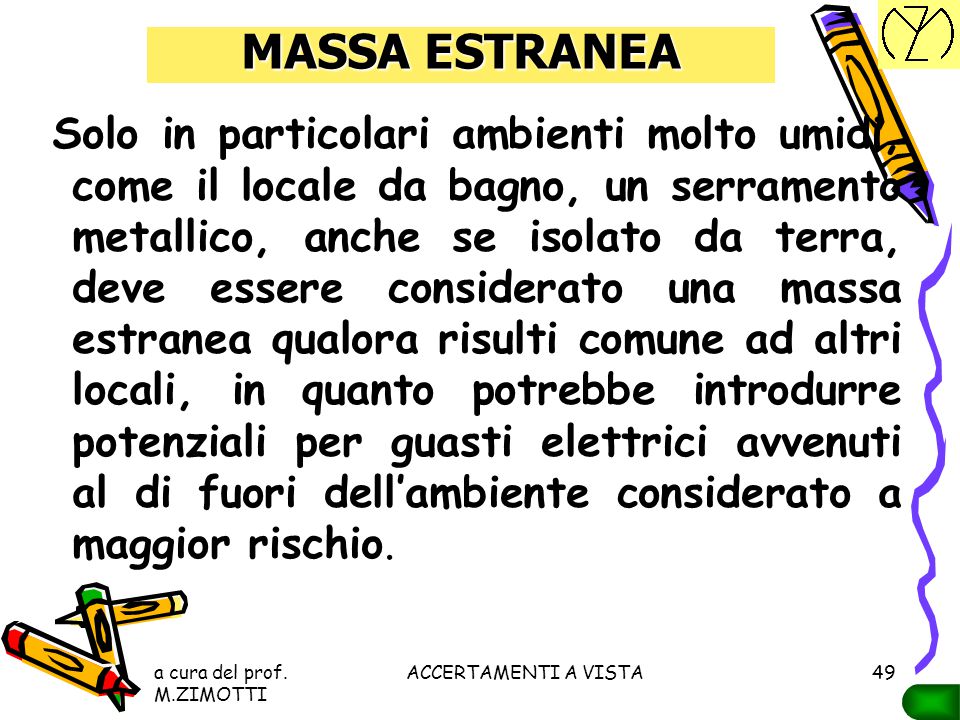The image features a predominantly white background, punctuated by a bold yellow rectangle at the top, containing the title "Masa Estranea" (spelled M-A-S-S-A-E-S-T-R-A-N-E-A). To the right, a cartoon-like depiction of a purple crayon or marker with an orange label draws a squiggly line extending down the length of the image. Beneath the title, a substantial block of black text, likely in Spanish, suggests an informational or educational context—possibly a PowerPoint slide for teachers, given the text's complexity. In the bottom left corner, a cluster of colored crayons (red, green, yellow) adds additional visual interest. The overall design, blending vibrant clip-art crayons with instructional text, indicates it may be part of a teaching resource or educational curriculum.